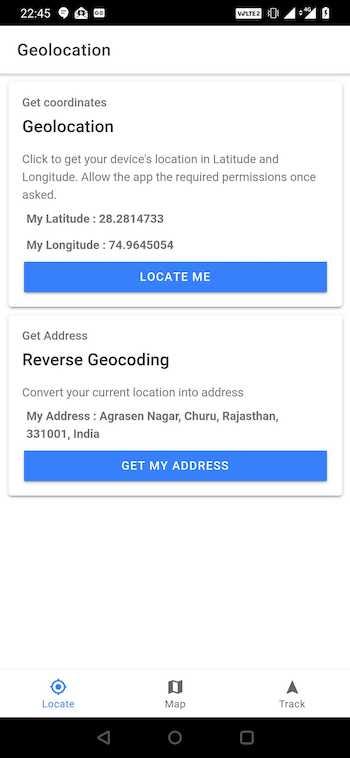A smartphone screenshot displays a geolocation app interface. At the top, a black bar reads "Geolocation." Below, a horizontal line separates the header from a square button labeled "Get Coordinates." The interface text states "Geolocation: click to get your device location" with fields for latitude and longitude. The current coordinates shown are latitude 28.281473 and longitude 74.9645054. Users are prompted to allow the app to require permission when asked by a button marked "Locate Me."

Further down, a white box offers options for "Get Address" and "Reverse Geocoding," which convert GPS coordinates into a readable address. Although the address is in India and challenging to pronounce, it's available upon request through the "Get My Address" button. At the bottom of the screen, additional options include "Locate," "Map," and "Track."